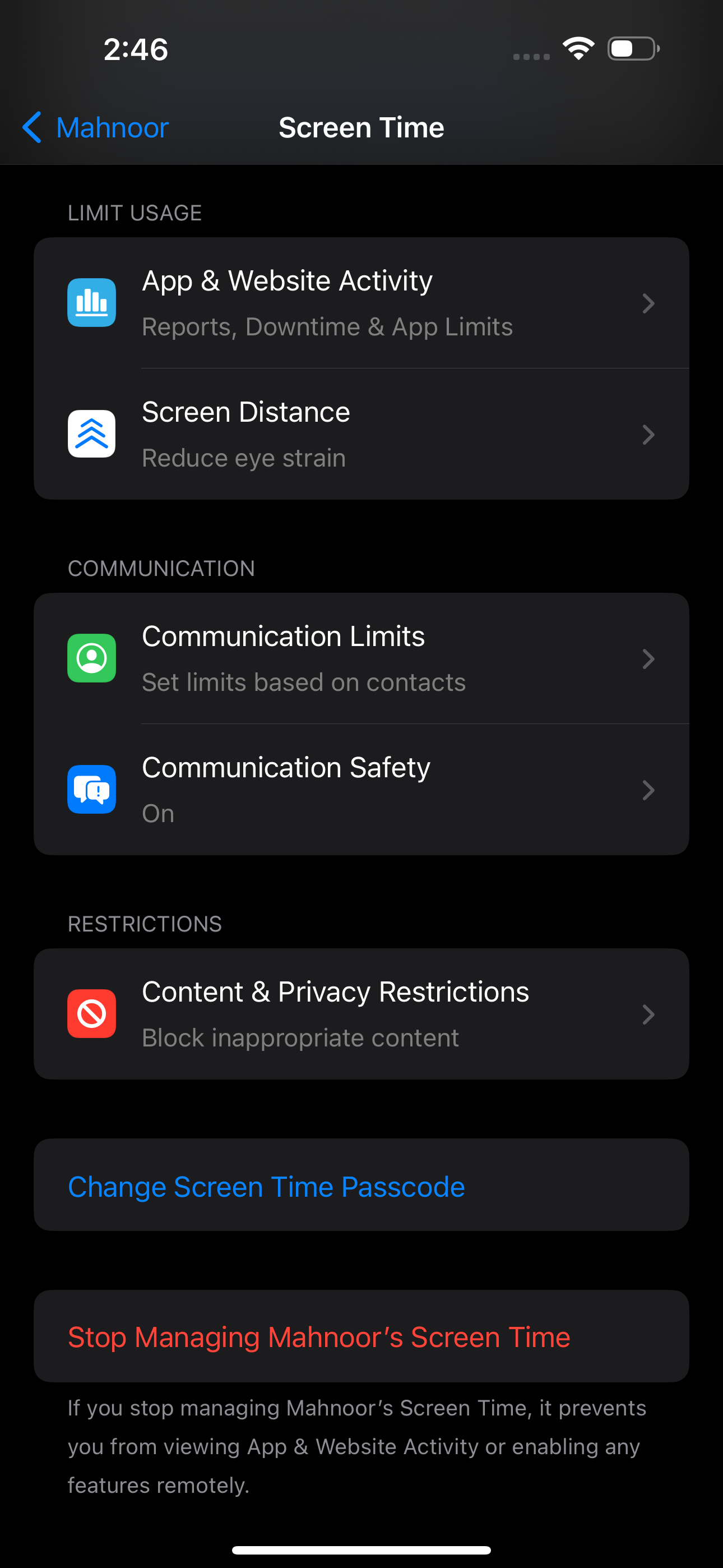The image shows a mobile phone screen displaying the "Screen Time" settings. The background is dark black, providing a stark contrast to the text and icons. At the top, we see the username "manure," presumed to be the owner of the device, along with a numerical identifier "246." Indicators for battery level and Wi-Fi connection are also visible.

The Screen Time settings are divided into several sections, each marked by colorful icons:

1. **Screen Time Summary** - A blue icon. This section includes options for limiting device usage, tracking app and website activity, and reporting app limits. There's a feature labeled "Screen Distance," symbolized by arrows pointing forward, designed to reduce eye strain.

2. **Communication** - This section is divided into:
   - **Communication Limits** - Identified by a green icon, this setting allows users to set usage limits based on contacts.
   - **Communication Safety** - Denoted by a blue icon with a message pop-up logo, this feature is currently turned on to ensure safe communication practices.

3. **Restrictions** - Marked with a red icon featuring a warning symbol, this section lets users enable content and privacy restrictions to block inappropriate content.

At the bottom of the screen, there's a button to change the Screen Time passcode and a red option that reads "Stop Managing Manure's Screen Time." Selecting this will prevent any remote monitoring or feature enabling for app and website activity. A white scroll bar is visible at the bottom, indicating that the user can navigate through more content in this menu.

This detailed layout provides a comprehensive overview of the screen time and communication safety settings on the device.